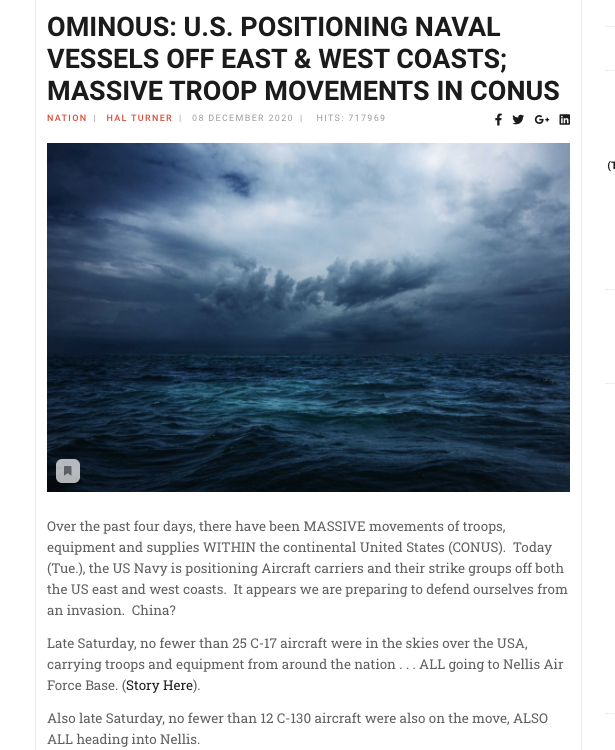Caption: 

"This image features an article titled 'Omnius: U.S. Positioning Naval Vessels off East and West Coasts; Massive Troop Movements in CONUS.' Written by Hal Turner and dated December 8, 2020, the article has accumulated 717,969 hits. Beneath the headline, there is a dramatic photograph of an ocean scene under stormy conditions. The sky is overcast with a break in the middle of the clouds, allowing a glimpse of light. The water below is turbulent and wavy, reflecting the intensity of the weather above. Below the image, a blurb reads: 'Over the past four days, there have been massive movements of troops, equipment, and supplies within the United States.'"